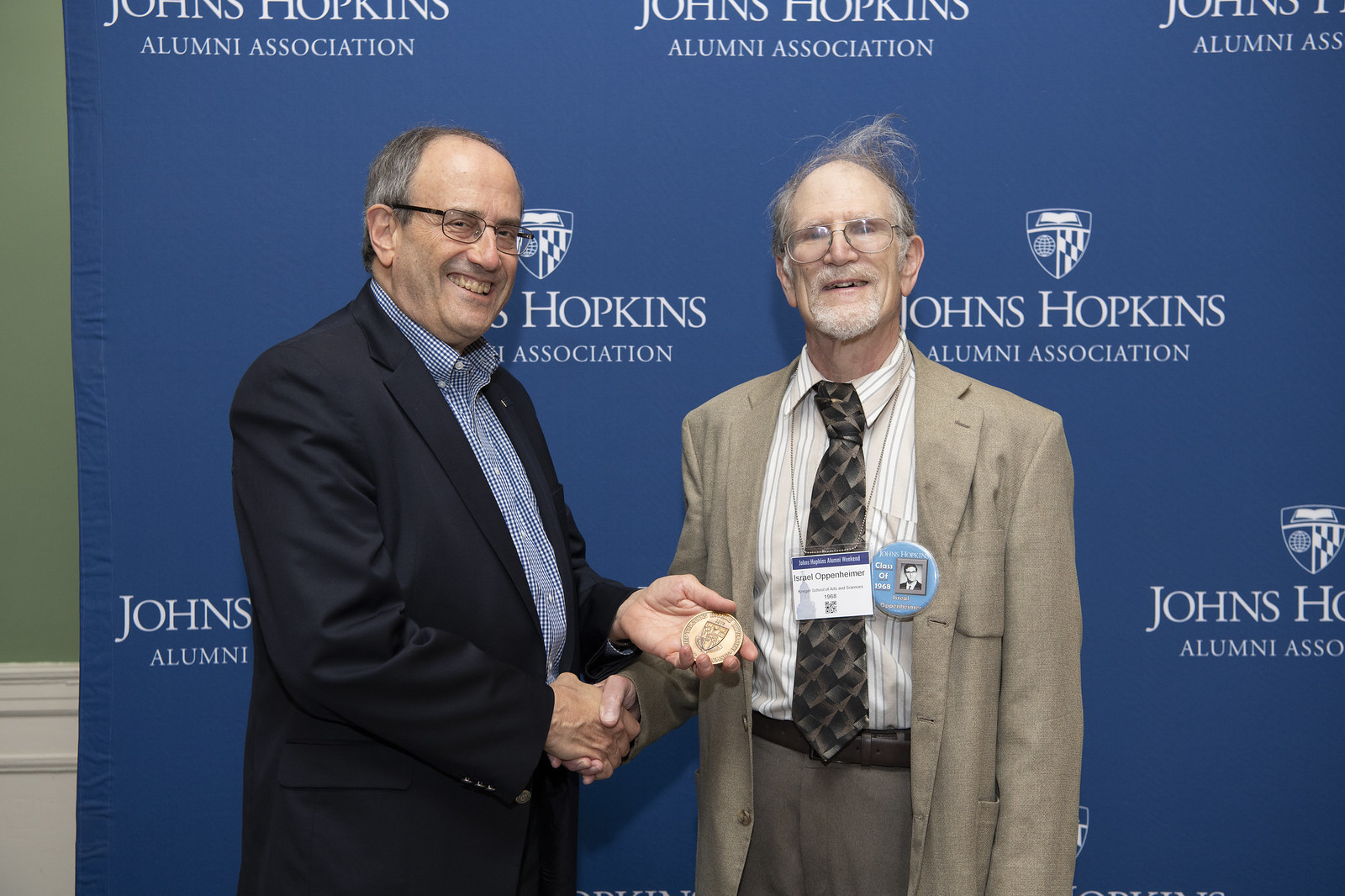In this detailed image from a Johns Hopkins Alumni Association event, two men are seen standing in front of a prominent blue banner featuring the Johns Hopkins Alumni Association logo, which includes the school's emblem — an open book atop a shield divided into regional symbols, including the Maryland flag pattern. 

The man on the left is middle-aged, clad in a dark blue suit with gold buttons adorning the sleeves over a blue and white checkered shirt. He is sporting glasses and has graying, salt-and-pepper hair. He is smiling and proudly holding a circular medal featuring the Johns Hopkins crest in his left hand. His right hand is engaged in a handshake with the second man in the photo.

This second gentleman is older, wearing a khaki tan blazer that seems slightly oversized paired with darker khaki pants and complemented by a brown belt. His outfit also includes a white and tan striped shirt and a fashionably eclectic tie displaying a blackish-grayish-tan pattern. He has glasses, somewhat disheveled hair with a noticeable tuft standing up and visible stubble across his jaw, suggesting a more casual appearance. The details suggest that this could be Mr. Israel Oppenheimer, a distinguished alumni from the class of 1968, possibly being honored with the medal presented by the man in the blue suit. The event appears to be both a celebration and a recognition of alumni achievements.